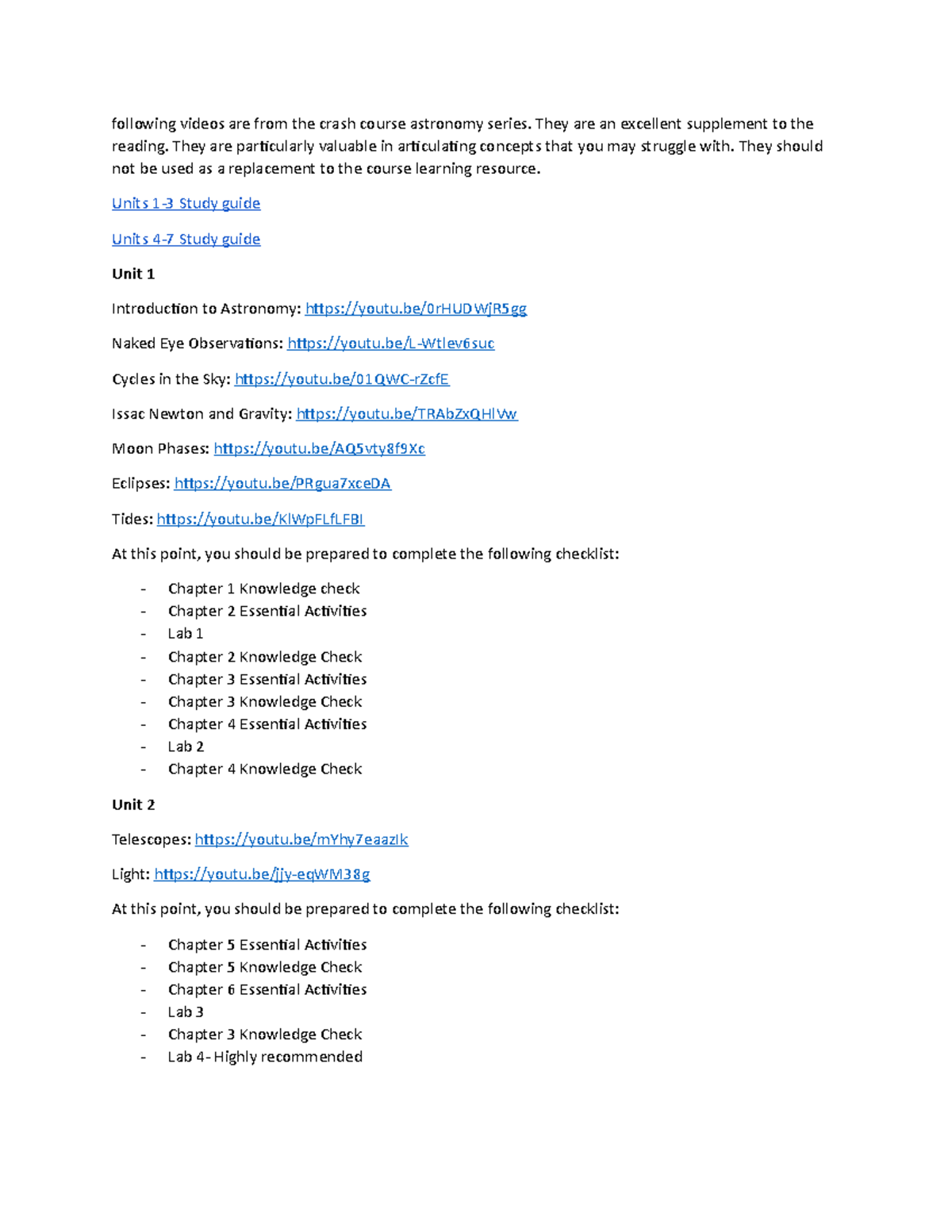**Detailed Caption:**

This image appears to be a screenshot featuring black and blue text at the top. The text serves as an instructional component, indicating: "The following videos are from the Crash Course Astronomy Series. They're an excellent supplement to the reading and provide valuable articulation of concepts you may struggle with. However, they should not replace the course’s learning resources."

The content seems to be organized as a study guide or set of chapter modules for an astronomy course. Listed under Unit 1 are several topics, each accompanied by a YouTube link:
- Intro to Astronomy
- Naked Eye Observations
- Cycles in the Sky
- Isaac Newton in Gravity
- Moon Phases, Eclipses, and Tides

Following these topics, it states, "At this point, you should be prepared to complete the following checklist," listing the chapter requirements as:
- Chapter 1: Knowledge Check
- Chapter 2: Essential Activities and Lab
- Chapter 3: Essential Activities and Knowledge Check
- Chapter 4: Essential Activities and Lab, Knowledge Check

Next, under Unit 2, it includes:
- Study of Telescopes with an accompanying YouTube video
- Light with an accompanying YouTube video

The text concludes with another checklist prompt: "At this point, you should be prepared to complete the following checklist," covering:
- Chapter 5: Essential Activities and Knowledge Check
- Chapter 6: Essential Activities and Lab
- Chapter 3: Knowledge Check and Lab 4 (highly recommended)

This structured layout suggests guidance for students to follow along with the provided multimedia resources, ensuring comprehensive coverage of the course material.